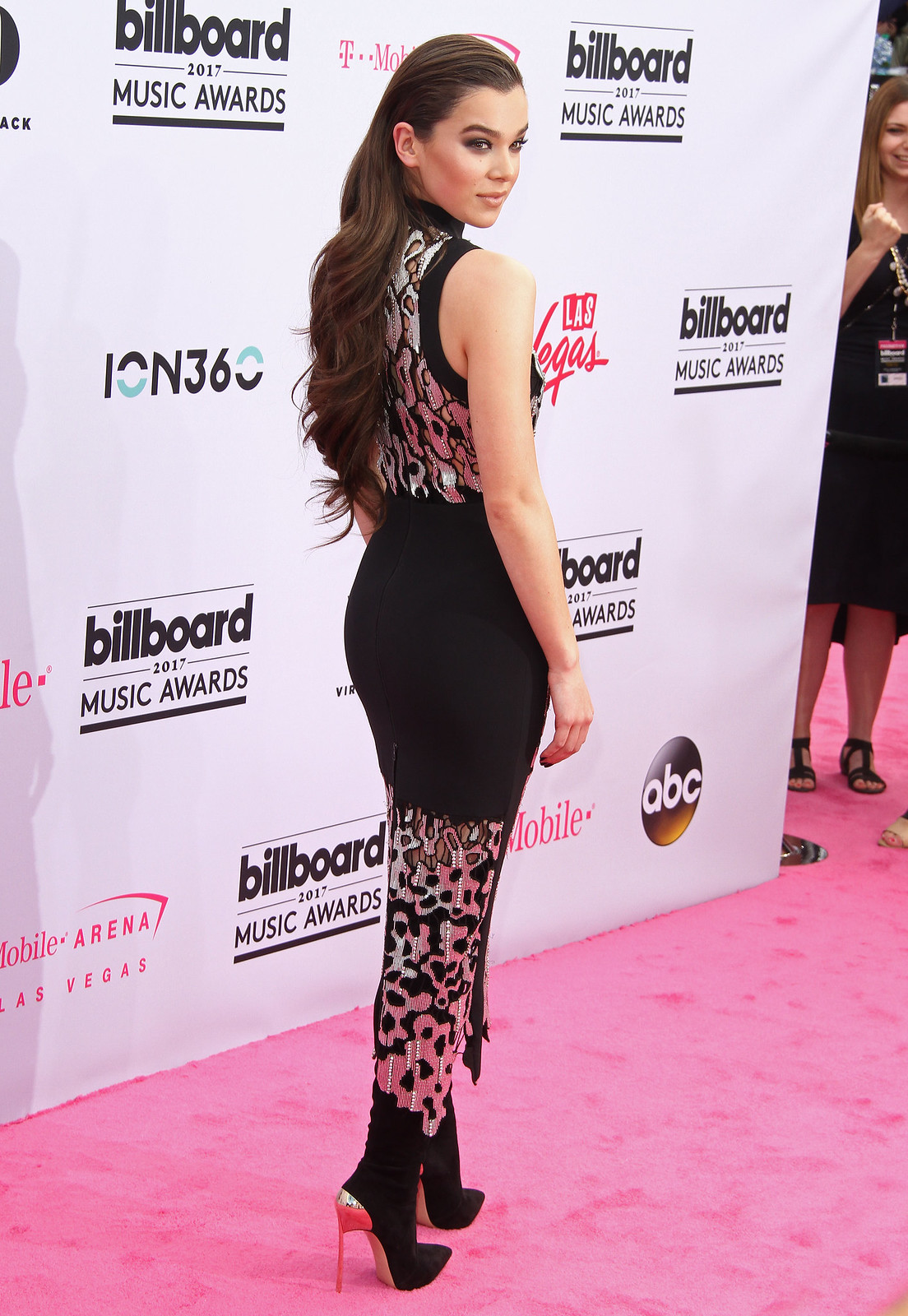The image depicts a vertically-oriented photograph of a woman posing elegantly on a pink carpet in front of a billboard at an event. The carpet extends diagonally from the bottom left to the right side of the image, leading up to the tall white billboard filled with repeated logos, including "Billboard 2017 Music Awards," "T-Mobile Arena Las Vegas" in pink, "ION 360," and the ABC logo in a black circle. The woman, with long, flowing brown hair reaching beyond her back, wears a striking one-piece dress with an intricate design. Her dress features a see-through black section around her waist and a silver, hole-patterned top and bottom, leaving her arms and shoulders bare. She stands confidently in tall black stiletto heels with shiny silver backs, looking back at the camera with grace.